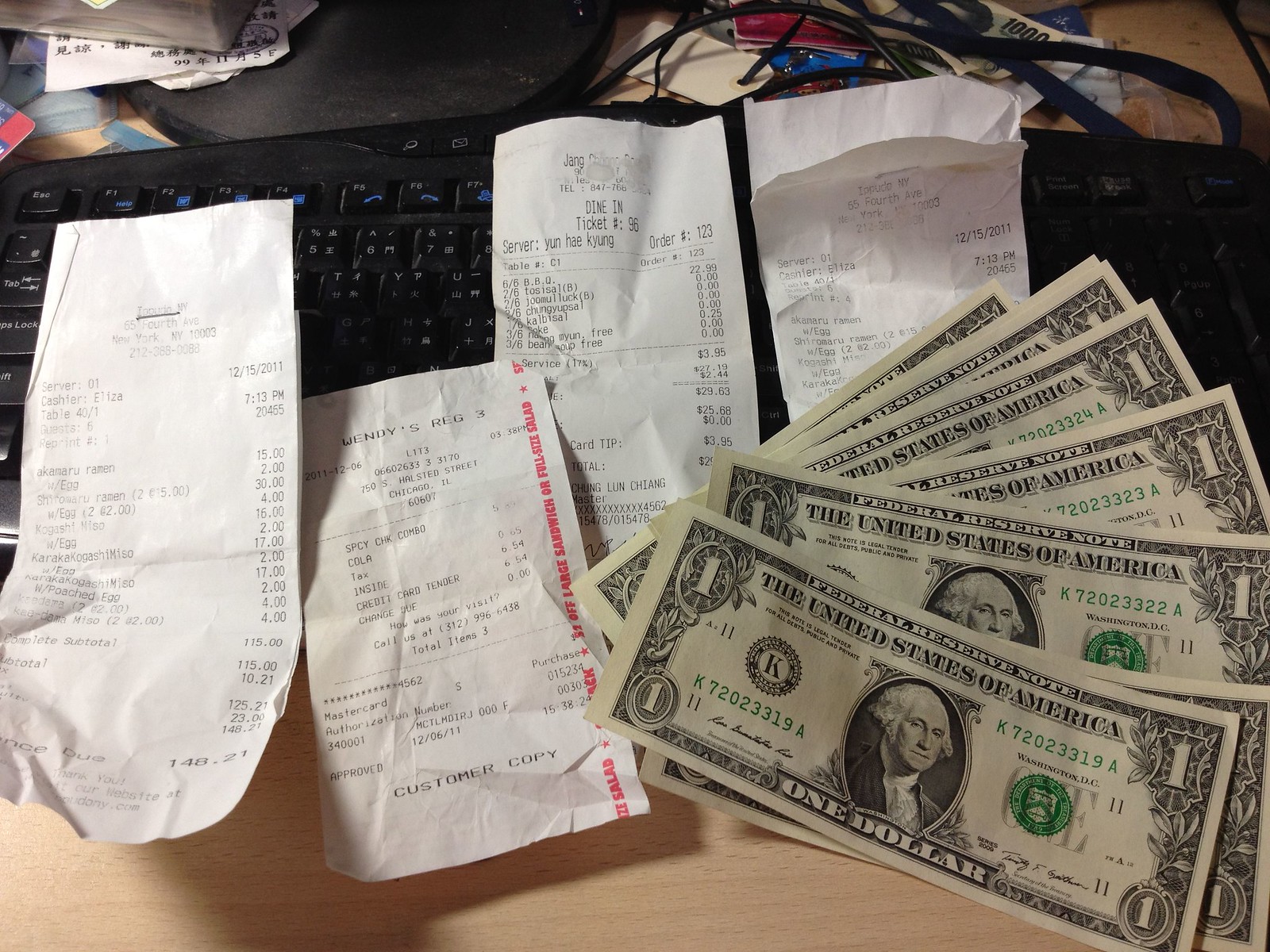The photograph displays a cluttered desktop scene with a black keyboard centered on a light wooden desk. Four white receipts with black print are spread across the keyboard, which also features a distinctive red print running up the right side of the second receipt. In the bottom right corner of the image, eight $1 bills are fanned out, forming an array amounting to $8. Behind the keyboard, various tags, cables, and papers are barely visible, suggesting a disorganized workspace. The close-up perspective captures the mundane details of what appears to be a personal accounting or expense-checking task, with receipts from different eateries like a ramen place and Wendy's adding context to the scene.